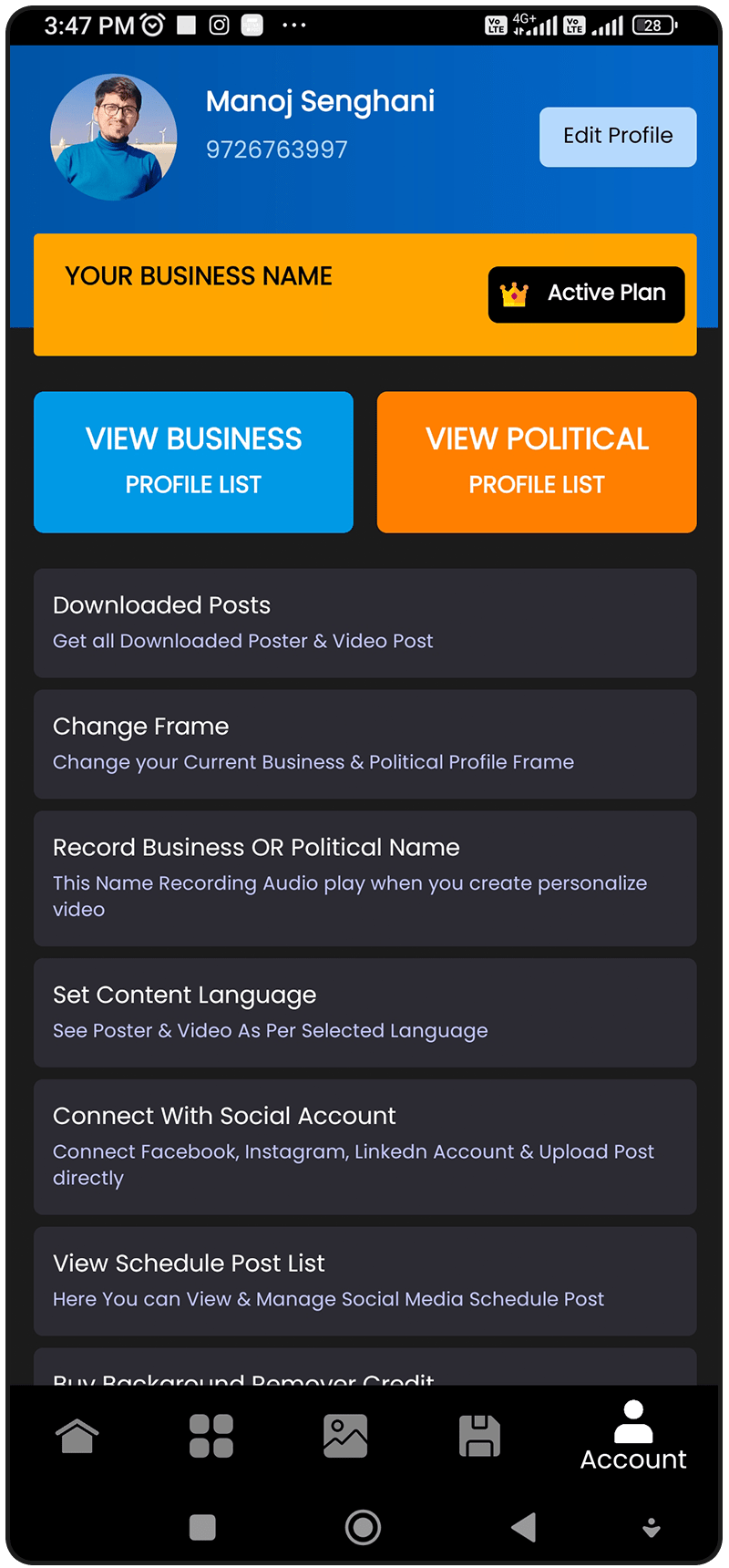This detailed business profile screen on a mobile application belongs to Minaj Singhani. The interface predominantly features a gray and black color palette with white text, accentuated by bright blue and orange buttons at the top. The presence of an "Edit Profile" button confirms that Minaj is logged into his account. His business name field is currently empty, indicating he has not yet established a business identity within the app. However, the screen indicates that he has an active plan with the program.

At the top of the screen, there is a series of functional buttons. One button allows Minaj to view his business profile and profile list. Adjacent to this is a conspicuous orange button labeled "View Political Profile List." Beneath these primary buttons, a series of secondary options are available for Minaj to interact with. These include access to his downloaded posts, the ability to change his frame, and the option to record a business or political name via audio.

Additionally, Minaj can set his content language preferences, connect the app to his social media accounts, and view a list of his scheduled posts. Further customization options lie in the app's settings section, where Minaj can navigate to the home screen, upload a picture, save his account details, or retrieve his account information.

The detailed screen view visible within the app on his phone provides a comprehensive overview of available functionalities and customization options, enhancing user experience for both business and political profile management.